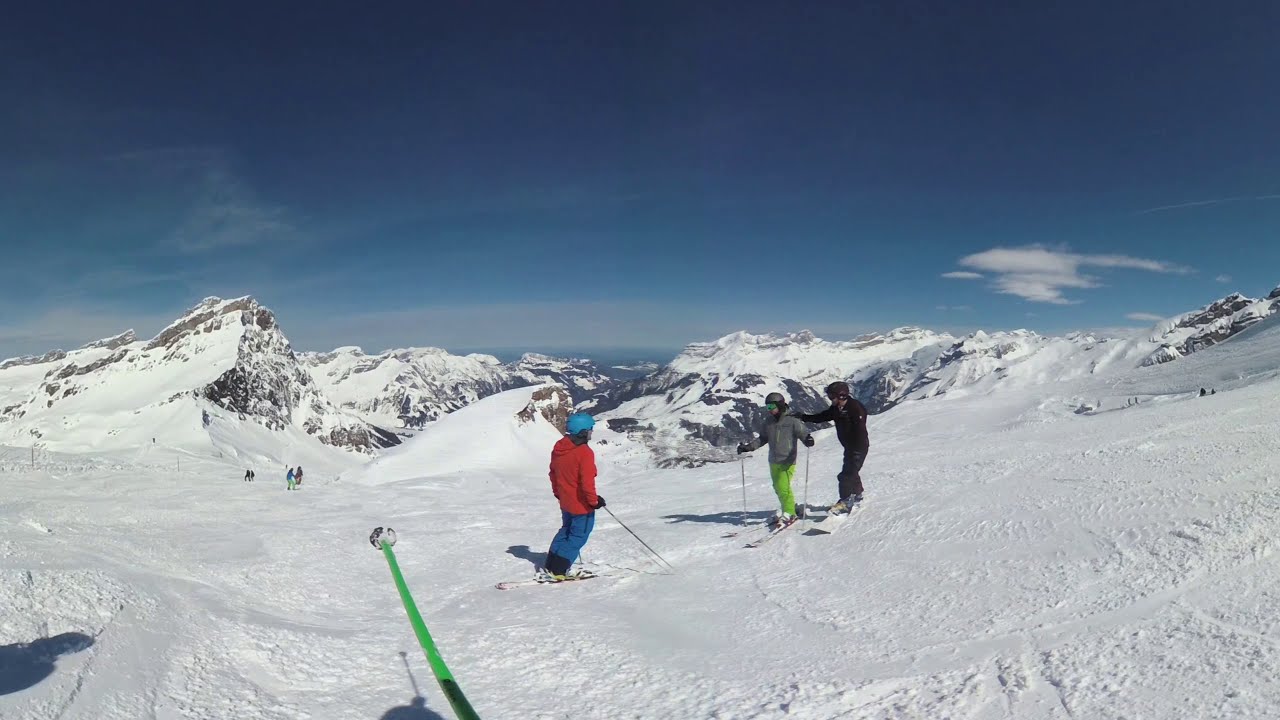On a sunny day with a bright blue sky and a few scattered clouds, a group of skiers is preparing to descend a snowy mountain slope. In the foreground, a skier, who appears in shadow, holds up one green ski pole, providing a unique perspective of the scene. At the center of the image, a person wearing a baggy red jacket, blue pants, and a blue helmet stands, facing slightly to the right toward another pair of skiers. This person, possibly a man or woman, is positioned prominently, indicating they might be a central figure or guide.

To the right of the central figure, a girl is seen wearing a gray jacket, gray helmet, and neon green pants. She has light blue glasses and seems to be in a welcoming stance with her arms partly outstretched, possibly initiating a hug. Beside her is a man, likely an instructor, dressed in all black gear. He is placing his hand supportively on the woman's shoulder, suggesting a moment of instruction or reassurance.

In the background, the expansive snow-covered mountains stretch out, adding depth and majesty to the scene. Farther down the slope, several other skiers are visible, enjoying the pristine conditions of the ski resort. The image beautifully captures the essence of a vibrant day in the mountains, teeming with the excitement and camaraderie of skiers ready to embark on their descent.